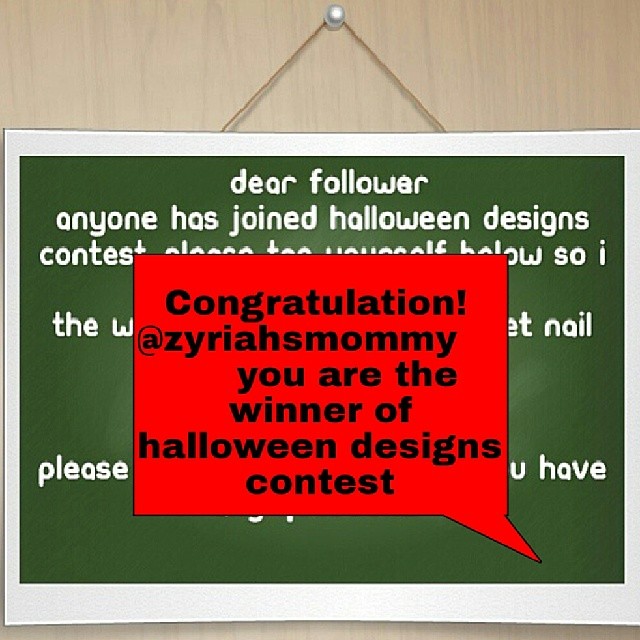The image features a computer-generated poster pinned to a wooden surface that appears greenish brown, with visible wood grain texture. The poster, which has a white rectangular border and a central green rectangle containing white text, is suspended from a brown string attached to a silver thumbtack. The readable part of the text says, "Dear Follower, anyone who has joined Halloween Designs Contest..." before being obstructed by an overlying red rectangular speech bubble with black text that reads, "Congratulations! At Zariah's Mommy, you are the winner of Halloween Designs Contest." The overall design looks somewhat haphazard, with the second red box obscuring the initial message, making it difficult to read the full original announcement.